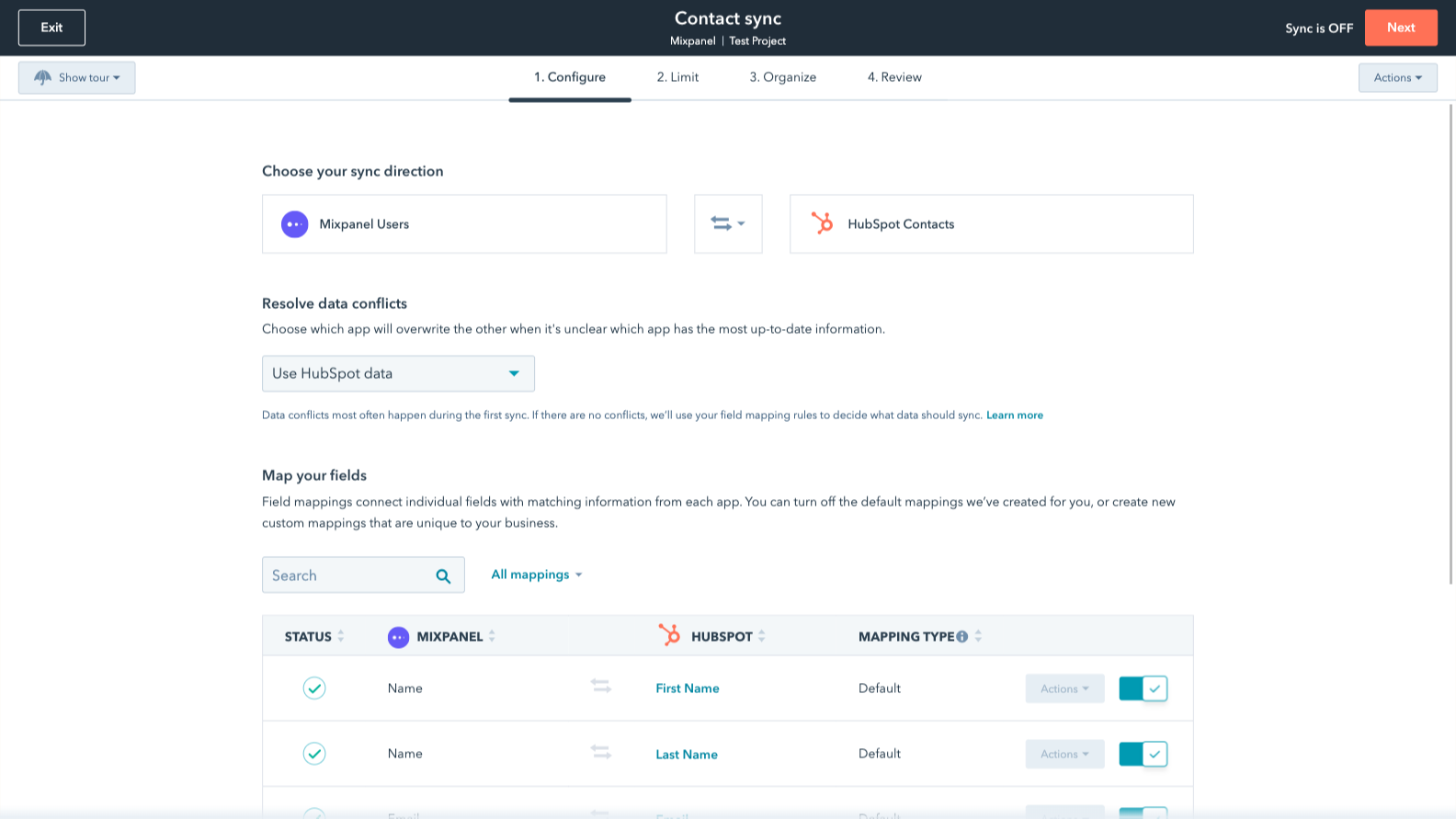This is a detailed screenshot of a web application interface for a contact synchronization process. At the top, the page is labeled "Contact Sync." Beneath this main title, there's a subtitle indicating "Mixpanel and Test Project." On the far left side of the screen, there is an "Exit" button. On the far right side, it indicates that the sync status is "Off," accompanied by an orange "Next" button.

Below this header area, an options toolbar is displayed. The first option includes a "Show Tour" button, which is represented with an umbrella icon and a drop-down arrow. Centrally located at the top of the screen, there are four sequential steps: "1. Configure," "2. Limit," "3. Organize," and "4. Review." The current view selected is "1. Configure."

Proceeding further down, the section titled "Choose Your Sync Direction" is presented. It offers two options: "Mixpanel Users" featuring a purple logo, and "HubSpot Contacts" with an orange logo, separated by left and right arrows and a drop-down menu.

The next area is "Resolve Data Conflicts," accompanied by a descriptive statement: "Choose which app will overwrite the other when it's unclear which app had the most up-to-date information." A drop-down box follows this, labeled "Use HubSpot Data," with an additional note: "Data conflicts most often occur during the first sync. If there are no conflicts, we'll use your field mapping rules to decide what data should sync," along with a "Learn More" button.

Following that, the "Map Your Fields" section appears, explaining that "Field mappings connect individual fields with matching information from each app. You can turn off the default mapping that we created for you or create new custom mappings that are unique to your business." This section includes a search bar labeled "Search" and a link on the right side saying "All Mappings."

Finally, detailed status columns are presented with headings "Status," "Mixpanel," "HubSpot," and "Mapping Type." Underneath, there are checkboxes labeled "Name," "First Name," "Default," and each of these fields includes checkboxes under the "Actions" column.

Overall, this screenshot thoroughly outlines the initial configuration and mapping process of syncing contacts between Mixpanel and HubSpot.